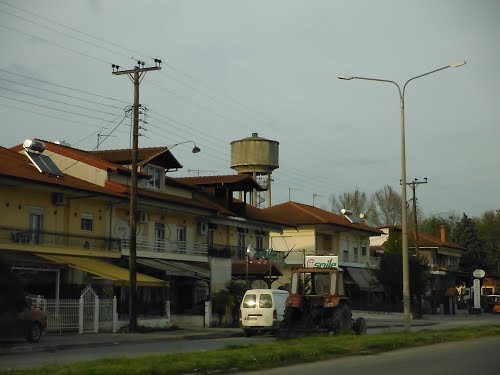The image depicts a small town or city street scene with an array of three-story buildings running from left to right. The closest building has sections of yellow and white with reddish-orange roofs, and the rooftop hosts solar panels on the left side. In front of this building, there is a white fence with pointed tops and a yellow awning aside from a silver-gray one. A white van with two back windows is parked on the side of the road, positioned next to a tractor marked with "SAIL" in green and a drawn face. The tractor is adjacent to a grassy median with a light pole emerging from it. Moving rightward, there are more buildings featuring a yellow structure with white walls and red roofs further down the street. Behind the buildings stands a dark gray cylindrical water tower. Power lines crisscross in front of these buildings, supported by numerous electrical poles. A street light with dual fixtures can also be seen sprouting from a pole. The background reveals a hazy, cloud-filled sky. Additional details include adjacent buildings with distinct features such as iron gates and balconies with white bars, another white building with solar panels, and a reddish-orange car. The furthermost building in the image is brown with a red roof, which appears near what resembles a gas station sign. Scattered trees add to the backdrop on the right.